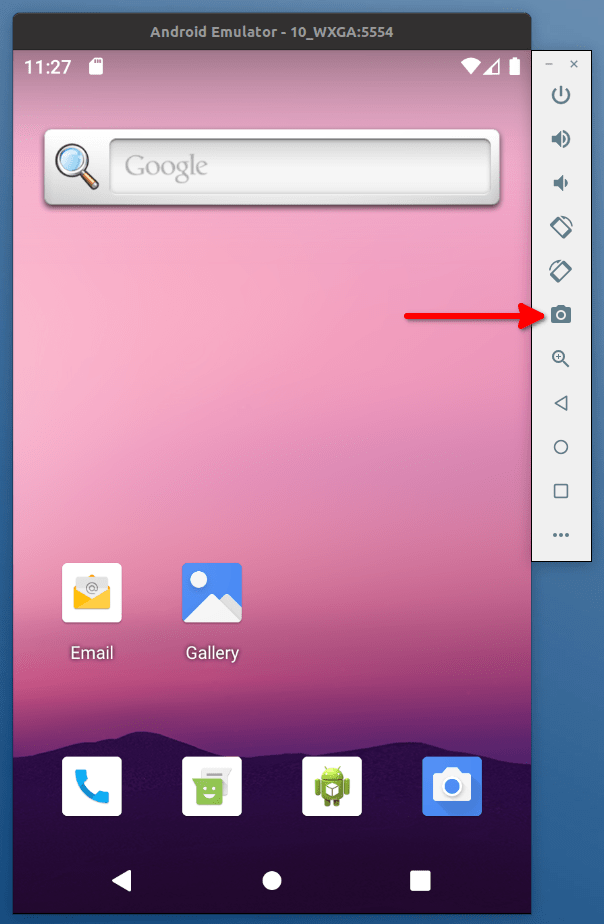Screenshot Description: 

The image captures a detailed screenshot of an Android smartphone's home screen. The background features a scenic mountain range under a serene pink sky, providing an aesthetically pleasing backdrop. Positioned at the top of the screen, a Google search bar offers quick access to online queries. The home screen hosts only two app icons: 'Email' and 'Gallery,' demonstrating a minimalist arrangement.

Prominently at the bottom, the standard Android menu bar includes icons for essential functions: a phone icon (calls), a chat icon (messages), an Android icon (app drawer), and a camera icon (camera access).

To the right of the main home screen is a translucent side menu with multiple functions. The menu includes icons for power, volume up, volume down, screen rotation controls, camera access, zoom in (plus sign), and navigation symbols like back, home, and a square (possibly recent apps).

A large, superimposed red arrow vividly points to the camera icon within this side menu, aiming to guide the user's attention towards the camera functionality available from this menu. This suggests that the screenshot is meant to instruct viewers on quickly accessing the camera through the side menu.